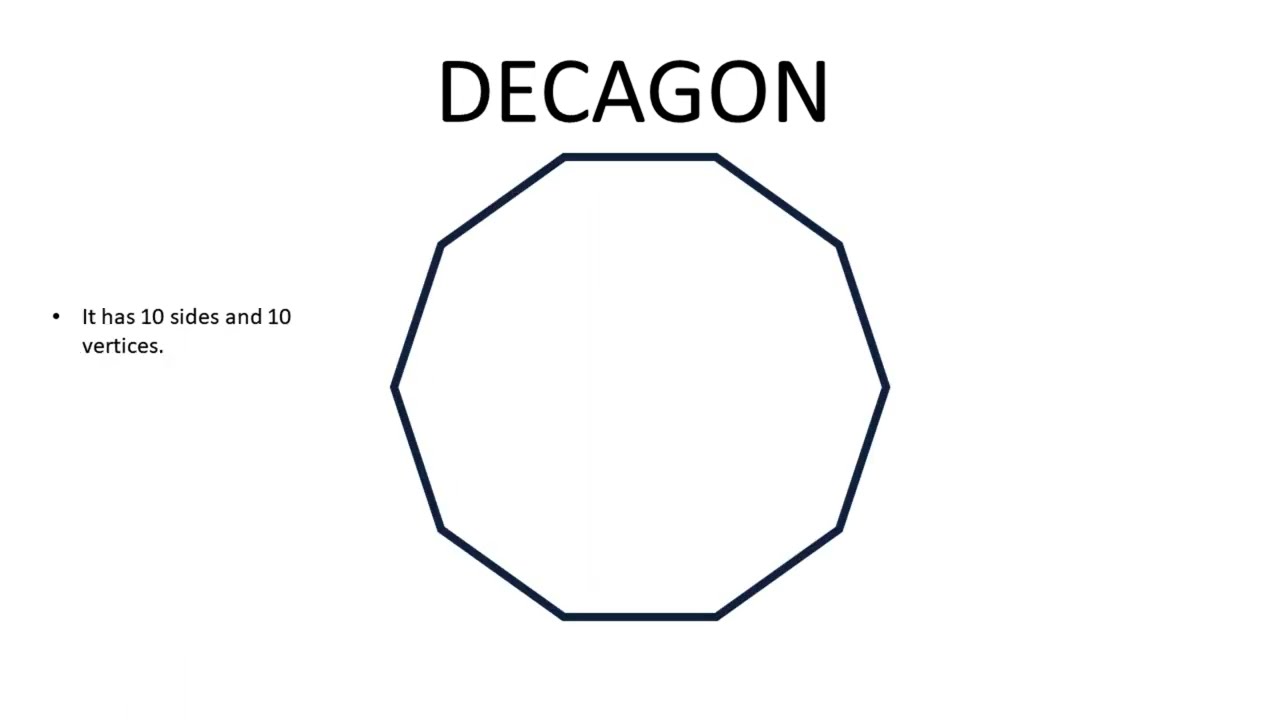The image features a detailed diagram set against a completely white background, which lacks any visible borders. Central to the image is a black-outlined decagon - a ten-sided polygon with all sides of equal length, measuring about an inch and a half to two inches both in height and width, with each side approximately half an inch long. Positioned at the top of the image in bold, black capital letters is the label "DECAGON." To the left of the diagram is a single small black bullet point, followed by the text "it has 10 sides and 10 vertices," also in black. Adding to the detail, a light gray horizontal stripe is present within the decagon, stretching from near the top to almost the bottom, with a smaller vertical stripe situated to the right of the horizontal one. This image appears to be an educational slide or informational card likely used in geometry classes to illustrate the characteristics of a decagon.